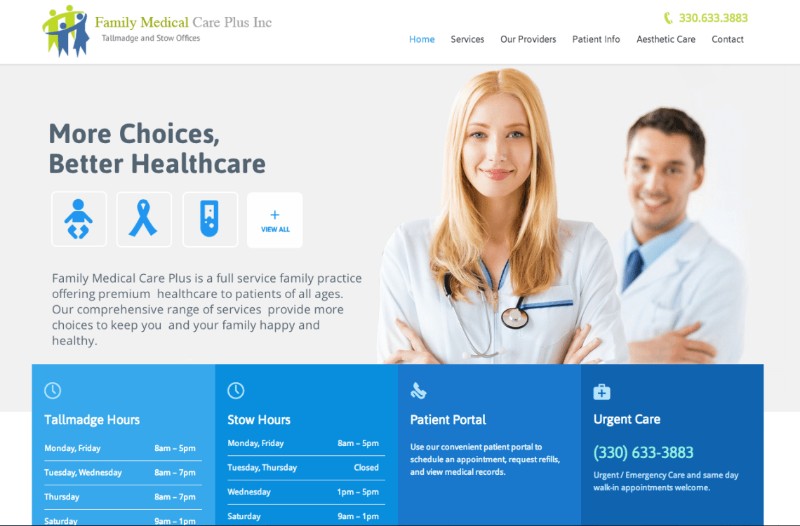Here we see a detailed screenshot of a computer screen displaying the website for "Family Medical Care Plus, Inc." The top section features a white border with the company name, "Family Medical Care Plus, Inc.," and a logo depicting two blue and two green figures holding arms in a circle, symbolizing unity and care. To the right, there's a phone number prominently displayed in green.

Below this header, the website offers six navigation tabs: "Health Services," "Our Providers," "Patient Info," "Aesthetic Care," and "Contact." 

Dominating the central portion of the screen is a large light gray rectangle that spans the width of the page. The right side of this rectangle features an image of two medical professionals. The forefront is a female doctor with blonde hair and a stethoscope around her neck, confidently looking at the camera. Just behind her stands a male doctor with short black hair, both of them smiling warmly at the viewer.

On the left side of this section, the phrase "More Choices, Better Health Care" is prominently displayed in bold text. Beneath this tagline, there are three icons followed by descriptive text in black, likely highlighting the key services or benefits offered by the facility.

At the bottom of the page, a wide blue border stretches across, divided into four sections with various shades of blue. Each section provides detailed information about the facility and its offerings, enhancing the user's ability to quickly grasp the essential features and services provided by "Family Medical Care Plus, Inc."